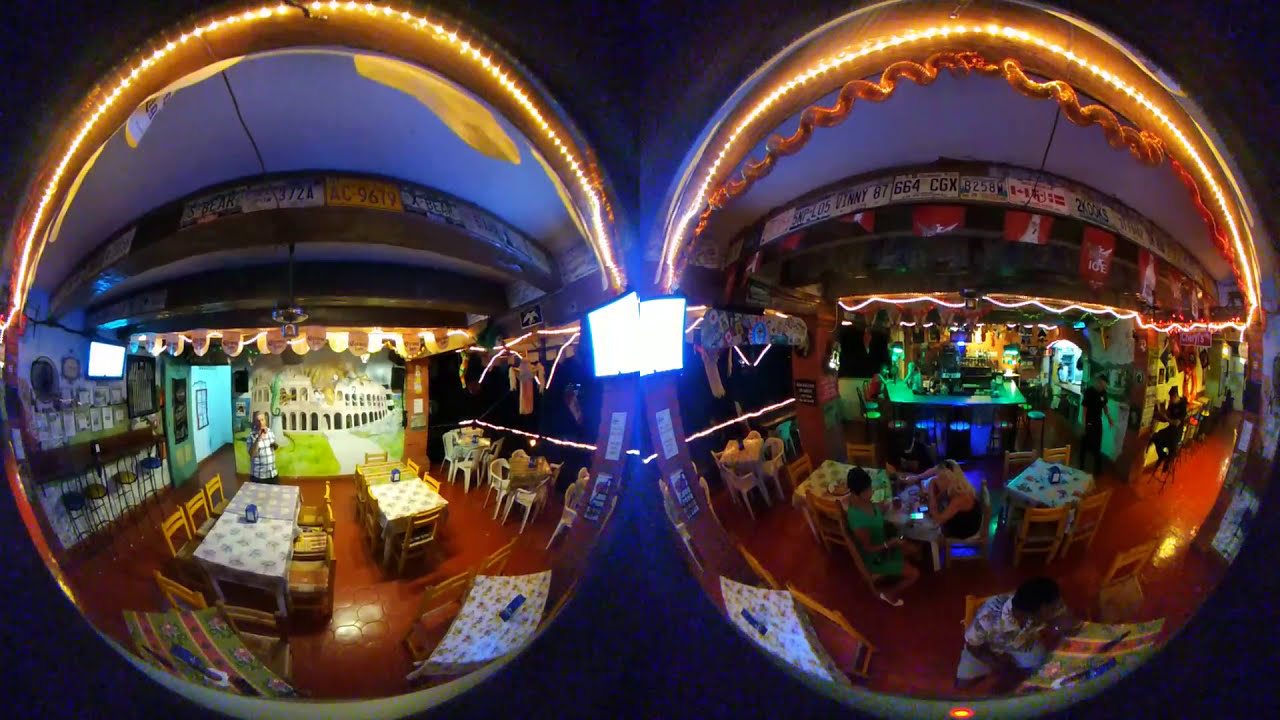The image depicts the interiors of a restaurant as viewed through two large, egg-shaped security mirrors, creating a slightly distorted, panoramic effect. The mirrors are centrally positioned and show two sections of what appears to be the same establishment with a hard tile floor. Both mirrors reveal a busy, colorful restaurant with multiple tables and wooden chairs arranged neatly in the center, and a bar area on the left side in the left mirror. Above, license plates are hung along what would be the ceiling. 

In the left mirror's reflection, there's a noteworthy piece of artwork or possibly a TV screen showing an image of a Roman or Greek building in the background, lending an Italian or Mediterranean ambiance. A man stands near one of the tables, and the overall scene is well-lit and vibrant.

In contrast, the right mirror's reflection is dimmer but equally detailed, showing additional seating and a central bar area surrounded by tables. The colors throughout range from black, yellow, blue, brown, red, orange, purple, light blue, gray to multiple shades of green, indicating a lively and diverse décor. Patrons can be seen, including a woman in a green shirt and a man in a white shirt, enhancing the bustling atmosphere of the restaurant.